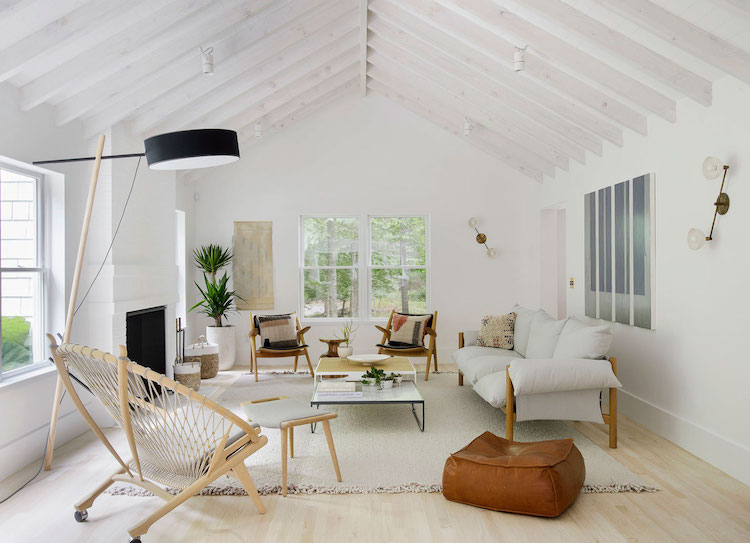This image features a modern, aesthetically pleasing living room characterized by its clean sight lines and open space. The room is predominantly white, boasting high arched ceilings with white wooden rafters and four white hanging lights. The floor is a light blonde wood, complemented by a cream-colored rug that spreads across the center of the room.

To the left, a fireplace is accessorized by a black lamp that extends outward. Nearby, an artificial plant in a white pot adds a touch of greenery. The main seating area on the right side includes a large grey sofa with multi-colored pillowcases, supported by light wood legs. Surrounding the sofa are several wooden chairs, including a distinct circular moon-shaped chair with rope detailing and another set endowed with cushions.

In the center of the room, two tiered coffee tables sit side by side, one featuring black metal edges and the other white metal with a brown middle. Adding to the comfort, a brown leather bean bag and what appears to be a brown ottoman are placed on the floor. The walls host four mirror-like pictures, enhancing the room’s spacious feel. A unique blonde wood floor lamp with a magnifying glass-shaped shade stands out, emphasizing the room’s blend of modern design with functional elegance.